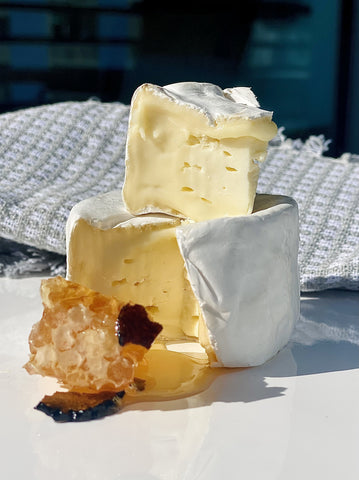This photograph features a beautifully arranged display of brie cheese on a white marble table surface. Dominating the foreground is a large wheel of brie cheese with a distinctive white rind. A large wedge has been cut from the wheel revealing its soft, gooey, yellow interior, and this wedge is artistically placed atop the wheel, forming a small cheese pyramid. The cheese’s interior is moist and opulent, with a slight drizzle of oil pooling at the base, highlighting its creaminess.

In the background, a neutral-patterned kitchen towel or tablecloth adds texture and subtle contrast to the scene. There is also mention of a hint of an orange, crystally object, possibly a piece of fruit or a snack, complementing the cheese's presentation. Blurred out in the farther background, one can glimpse doors and windows, completing the rustic yet elegant setting.